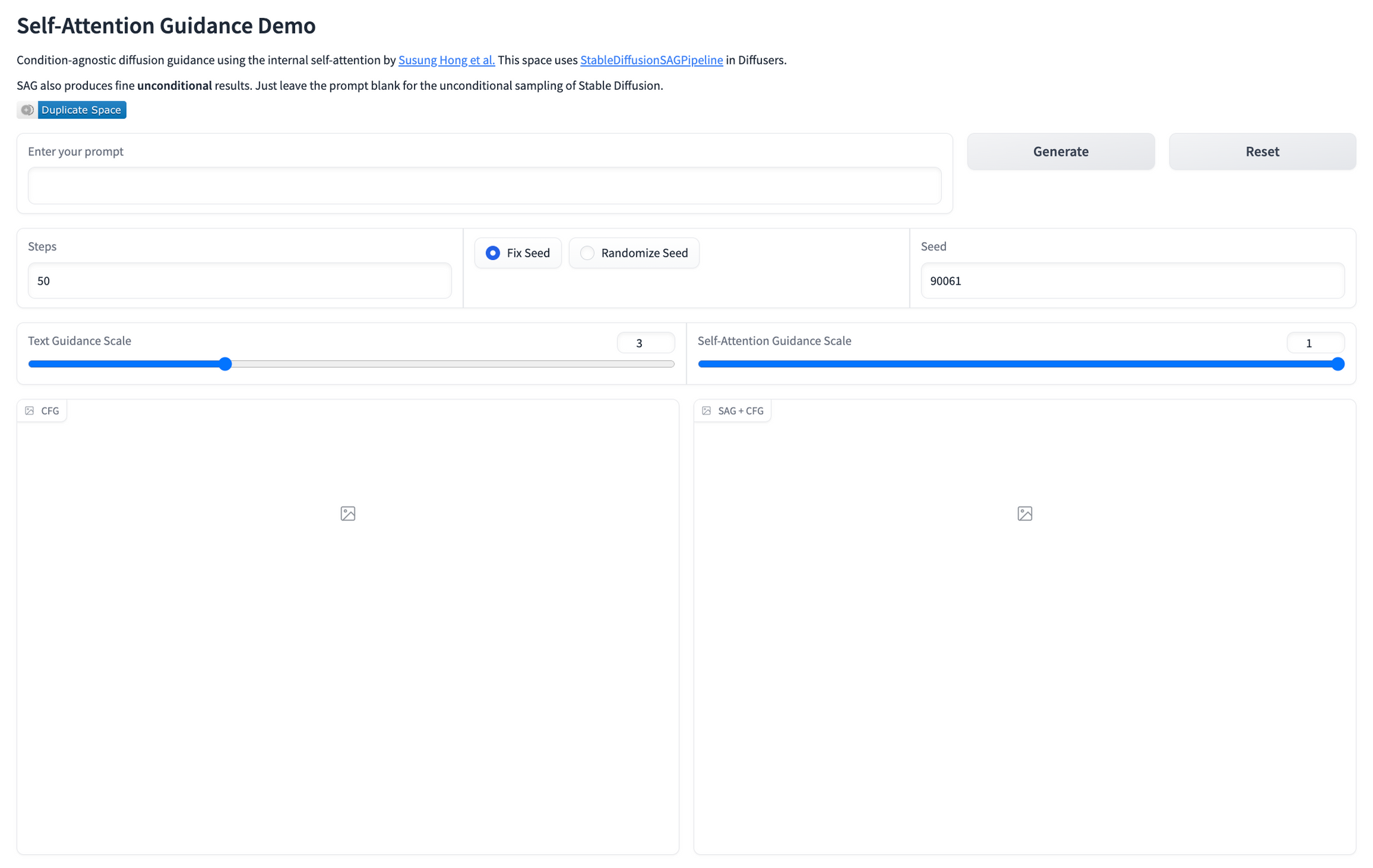This image showcases a computer application titled "Self-Attention Guidance Demo," which is prominently displayed at the top left corner. Below the title, there is a subtitle reading "Condition Agnostic Diffusion Guidance using the Internal Self-Attention by Suseong Hong et al." This application pertains to the "Stable Diffusion SAG Pipeline" and "Diffusers." It is noted that SAG can generate fine unconditional results by leaving the prompt blank during the unconditional sampling of stable diffusion.

In the main interface, there is a text box labeled "Enter Your Prompt," which is currently empty. Adjacent to this, on the right, are two gray buttons labeled "Generate" and "Reset." 

Further down, there are several interactive fields and controls. A text box labeled "Steps" is set to 50. Next to this are two button options: "Fix Seed" and "Randomize Seed," with "Fix Seed" being selected. The "Seed" text box contains the value "90061." 

The interface also includes two slider scales. The "Text Guidance Scale" is filled approximately one-fourth of the way, while the "Self-Attention Guidance Scale" is completely filled.

Toward the bottom of the application, there are two separate gray boxes, outlined by lines and each containing a small gray image icon in their centers, indicating placeholders for images that have not been generated yet.